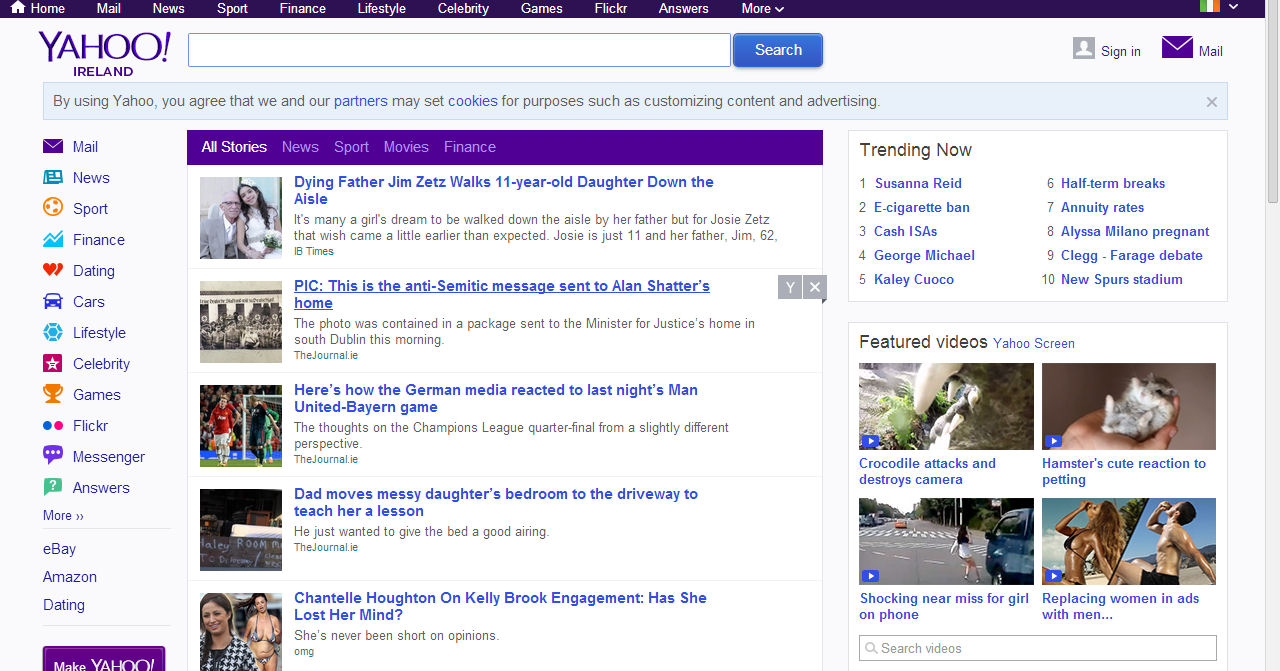The image displays the Yahoo! Ireland homepage featuring a classic, older-style Yahoo design. The interface is characterized by a white background and a distinctive purple bar running horizontally across the center of the page. The page is populated with various sections and panels.

On the left pane, there are categories including Mail, News, Sports, Finance, Dating, Cars, Lifestyle, Celebrity, Games, Flickr, Messenger, Answers, eBay, Amazon, and Trending Now. A prominent box showcases trending stories with featured videos displayed in a series of squares.

Amid the collection of news snippets and links, the design highlights elements typical of the era's web aesthetics. The overall layout remains uncluttered, dominated by the simplicity of a white backdrop. Contributing to a nostalgic atmosphere, this Yahoo! homepage snapshot serves as a reminder of early internet browsing experiences.

The caption also includes some repeated personal anecdotes emphasizing the qualities of a woman described as "a hard worker" and "a really good mom," underscoring her friendly, helpful, and outgoing nature.